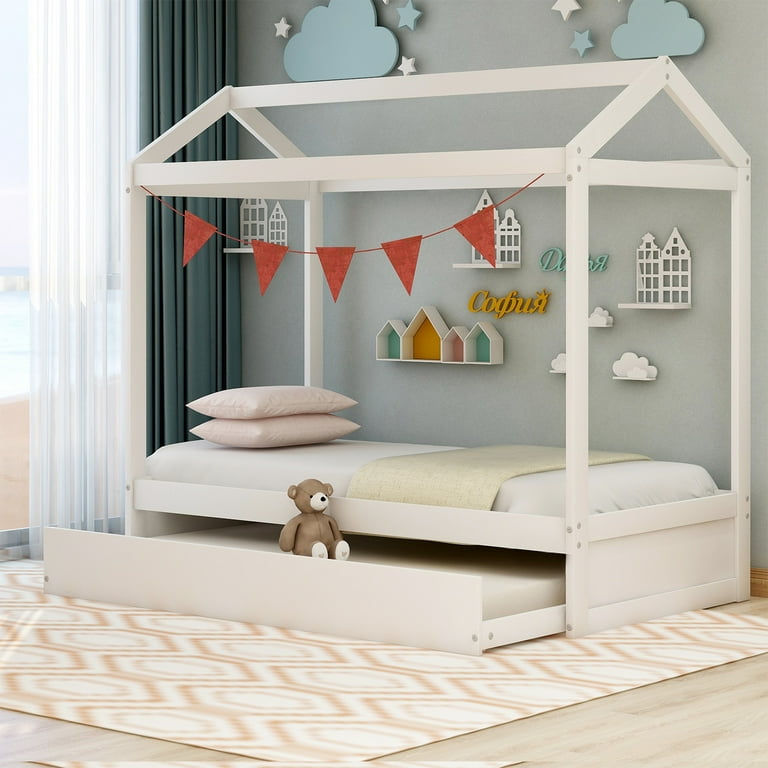The child's bedroom in the photograph appears meticulously arranged, potentially as part of a Target magazine or advertisement. A small white bed, with a house-shaped wooden frame mimicking the structure of a barn, occupies the foreground. The bed includes a pullout drawer beneath, which holds a brown teddy bear. The bed is neatly made with white sheets, a cream-colored blanket, and two pink pillows at the end. A green blanket is also neatly folded on top of the bed. The back wall, painted a soothing light gray, is adorned with playful decorations including cutouts of clouds, stars, buildings, and house-shaped shelves. Additionally, a string of red pennants adds a splash of color above the bed frame. To the left, sunlight streams through a window dressed with white and green curtains. The room features a blonde wood floor accented by an orange and white geometric-patterned rug, completing the cozy yet styled ambiance.